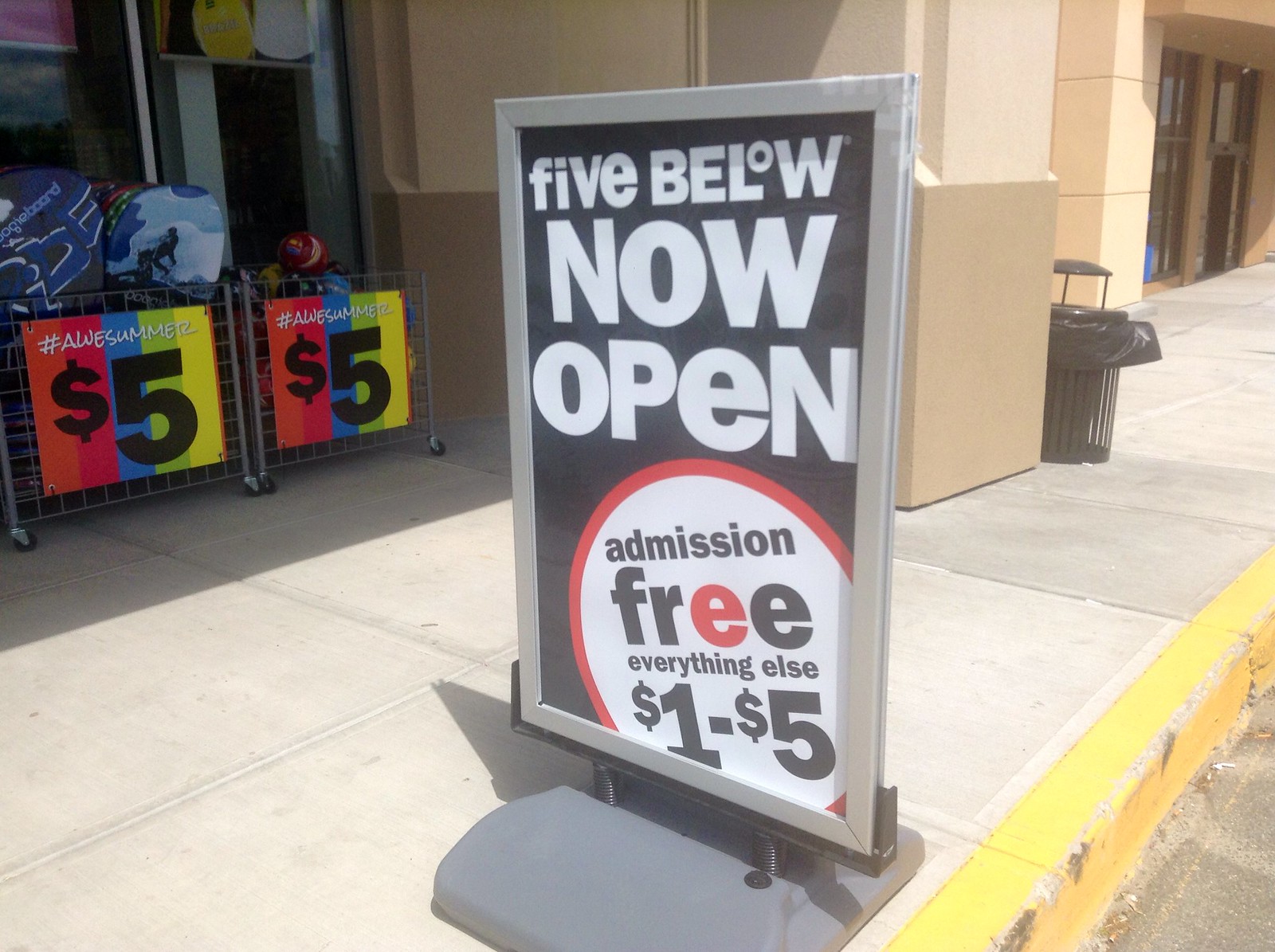This is a color photograph taken outdoors on a sunny day, showcasing a sidewalk scene centered around a sign for the store Five Below. The main sign, set in a silver frame on a gray pedestal with a black spring base, features a black background with white text that reads "Five Below" at the top, followed by "NOW OPEN," and below that, a white circle with the text "Admission Free," where the first 'E' in "Free" is red, and "Everything else $1 to $5."

The setting is a concrete sidewalk with a yellow-painted curb visible in the lower right corner. The store's entrance is situated behind the sign, with doors and additional storefronts seen further down the walkway. Adjacent to the sign, two store bins displayed outside are filled with summer items like flip-flops, beach toys, and balls, each marked with multicolored square signs that say "$5" and "#AWESOME" in large black font. The lower half of the store building is dark tan, transitioning to light tan above.

In the broader scene, further down the sidewalk to the right, there is a trash can with part of a trash bag hanging out. The bright sunlight casts clear shadows on the sidewalk, creating a lively and inviting atmosphere.